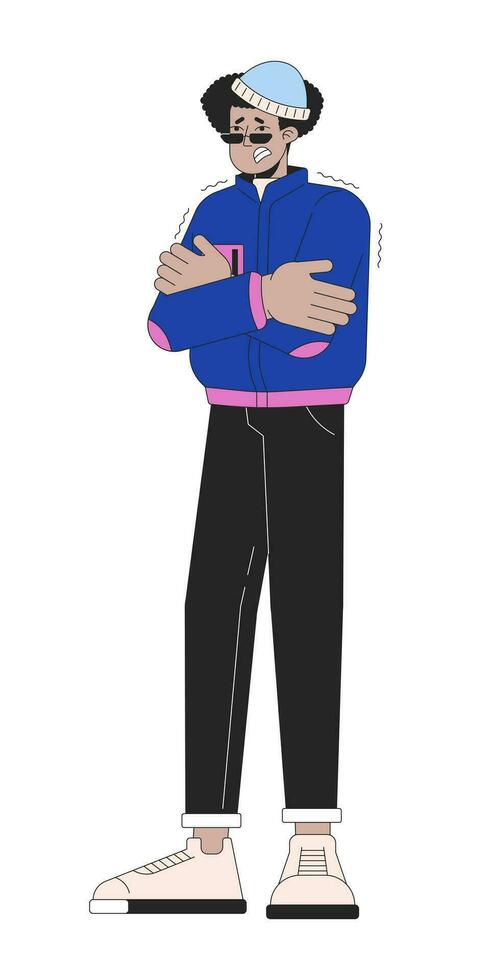This image is a cartoon depiction of a light brown-skinned man standing slightly to the left, set against a white background. He appears to be cold, demonstrated by his arms crossed tightly over his chest and the wavy black lines around his shoulders and upper arms indicating shivering. He has a concerned look, with raised eyebrows and chattering teeth. The character is adorned in black sunglasses perched at the end of his nose, revealing his dark eyes, and a light blue beanie with white trim sits atop his black afro hair. He is dressed in a blue jacket with pink trim, long black pants with white cuffs, and off-white sneakers with black soles. His ankles and hands, not covered by socks or gloves, expose his light brown skin, further emphasizing his cold state.